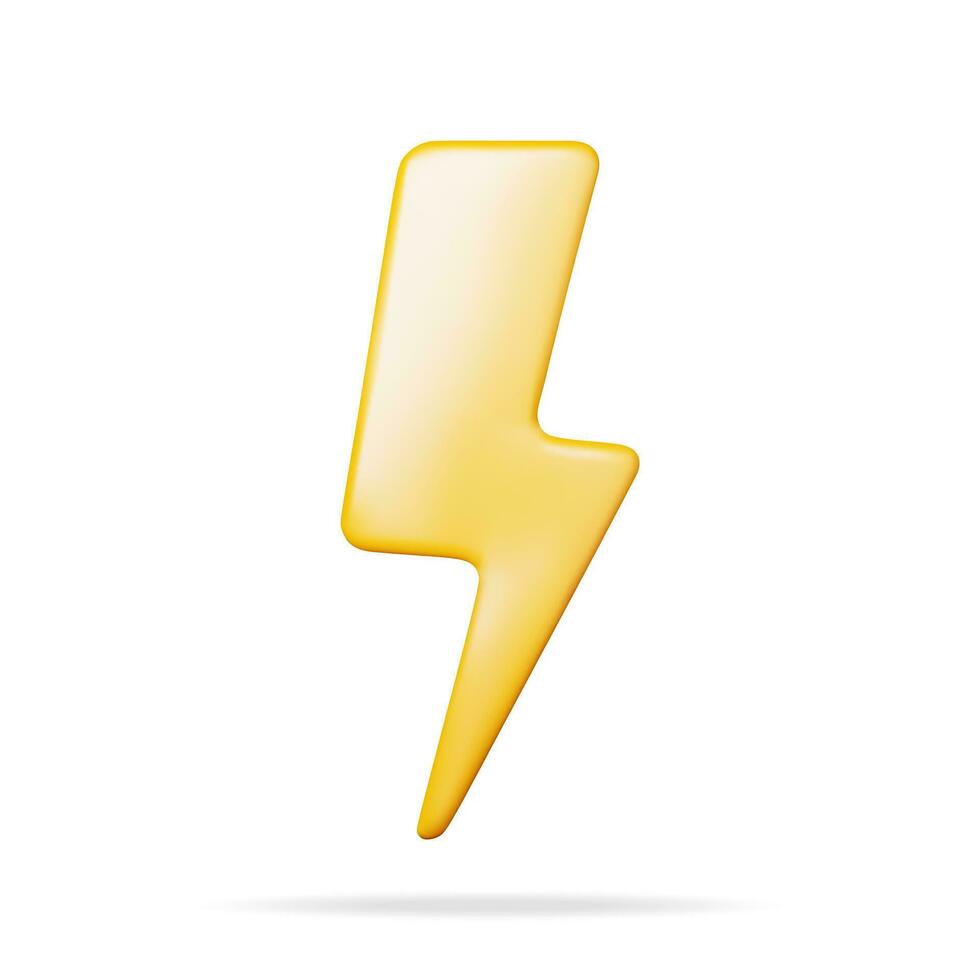This computer-generated image features a cartoon-like, light yellow lightning bolt with a slight 3D texture, achieved through varying shades of yellow, creating lighter spots that simulate light reflection. The lightning bolt, which starts at the top right, angles left, right, and left again before tapering into a triangular tip, appears to hover above the bottom of the completely white background. The darker yellow outline accentuates its shape, while a shadow beneath it emphasizes its floating look. The simplicity and design of the lightning bolt, with its 5 points and three-dimensional appearance, make it resemble an emoji or a graphic from a children's TV show.